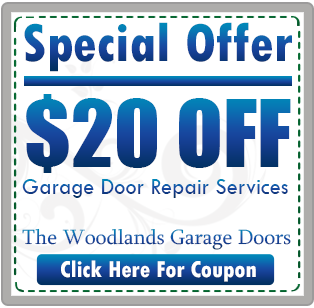Detailed Description: 

This image presents a digital coupon with a clean, newspaper-like design. At the top, "Special Offer" is prominently displayed in a gradient blue text, which transitions from a lighter sky blue to a deeper navy blue. A bold horizontal blue line separates this header from the main content below.

The central focus of the coupon is the bold offer text "$20 OFF," also in a gradient blue. Beneath this, in smaller blue font, are the words "Garage Door Repair Services" followed by "The Woodlands Garage Doors."

A striking call-to-action is centered in the lower portion of the coupon, with the words "Click Here for Coupon" written in white, set against a solid blue background. This text also features a blue gradient, mirroring the one used above.

The entire composition is set against a white background, adorned with a subtle light-gray motif, possibly a fleur-de-lis or a similarly intricate design. Encasing the content is a dotted line border, giving the digital coupon the visual appeal of a traditional paper coupon meant to be cut out. The outermost edge of the image is defined by a solid gray border.

This digital coupon effectively merges modern interactivity with a classic newspaper or magazine coupon style, appealing to users through its familiar and inviting design.